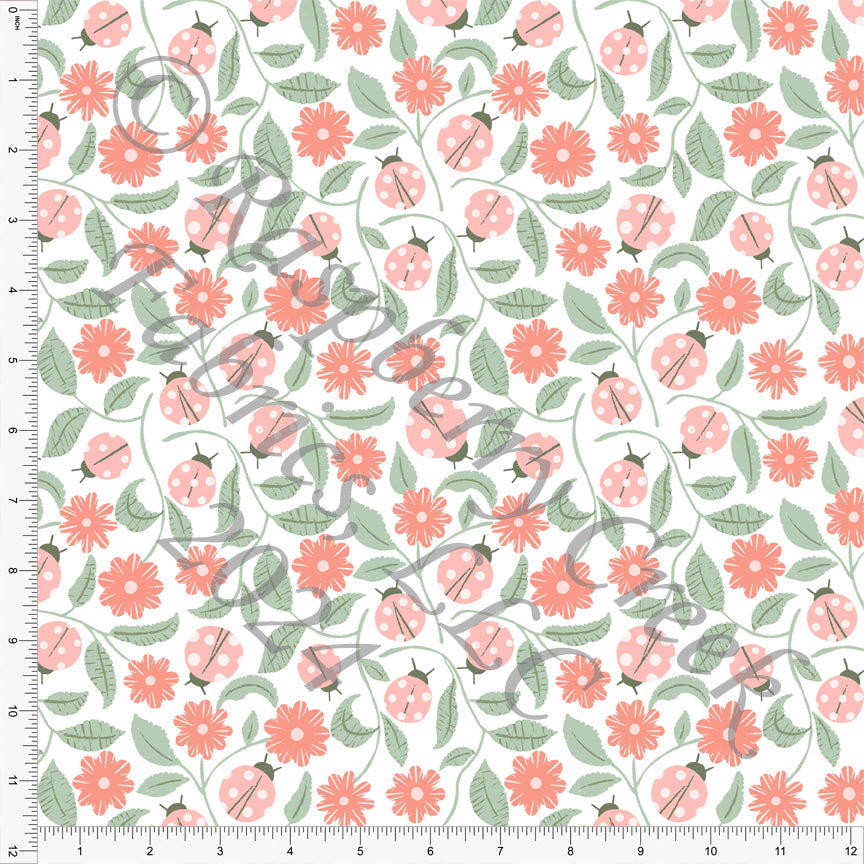The image depicts a square foot sample of wallpaper or fabric with a repeating floral pattern. The design includes pastel green leaves, pastel pink ladybugs with white spots, and darker pink or red flowers. A white background enhances the overall clarity of the pattern. Superimposed diagonally across the image is the text "Raspberry Creek Fabrics, LLC, 2024," indicating the copyright. Along the left and bottom edges of the image are foot-long rulers marked in inches from 0 to 12, which help to measure the sample’s dimensions. The bright setting highlights the detailed and colorful elements of the pattern.